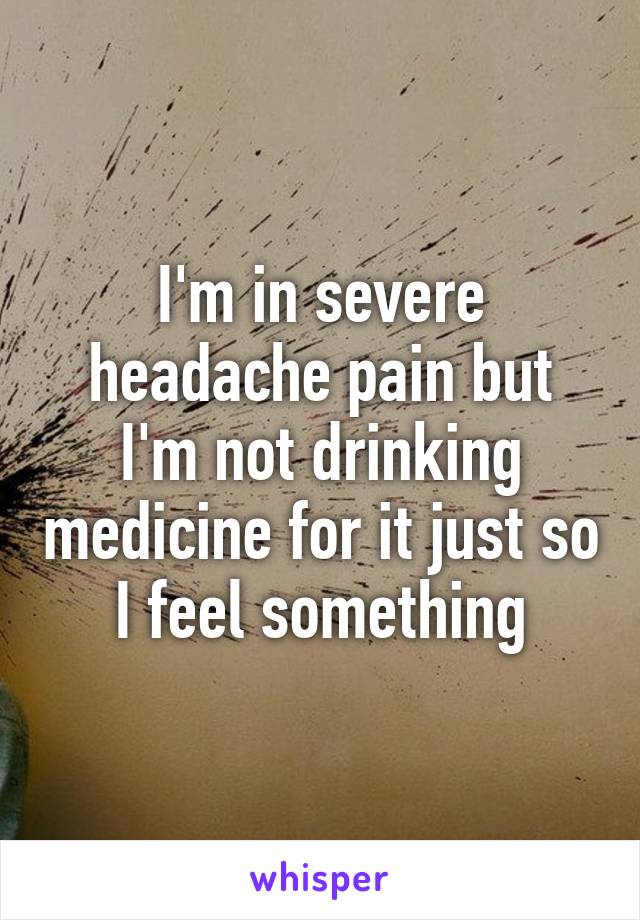The image depicts the aftermath of a violent event, implied by dark red and black spatter concentrated on the middle right and dispersed across the background, which is a tan-colored, taupe wall. The chaotic pattern of the spatter, with some darker streaks, evokes the sense of a tumultuous, swirling journey, much like navigating through a snowy vortex. On the bottom left corner, there appears to be the faint image of a light blue shirt or part of someone's shoulder. The focal point of the image is a caption in a white, sans-serif font that reads, "I'm in severe headache pain but I'm not drinking medicine for it just so I feel something." Below this statement, at the bottom of the image, is a white color block containing the word "whisper" in all lowercase, purple font.